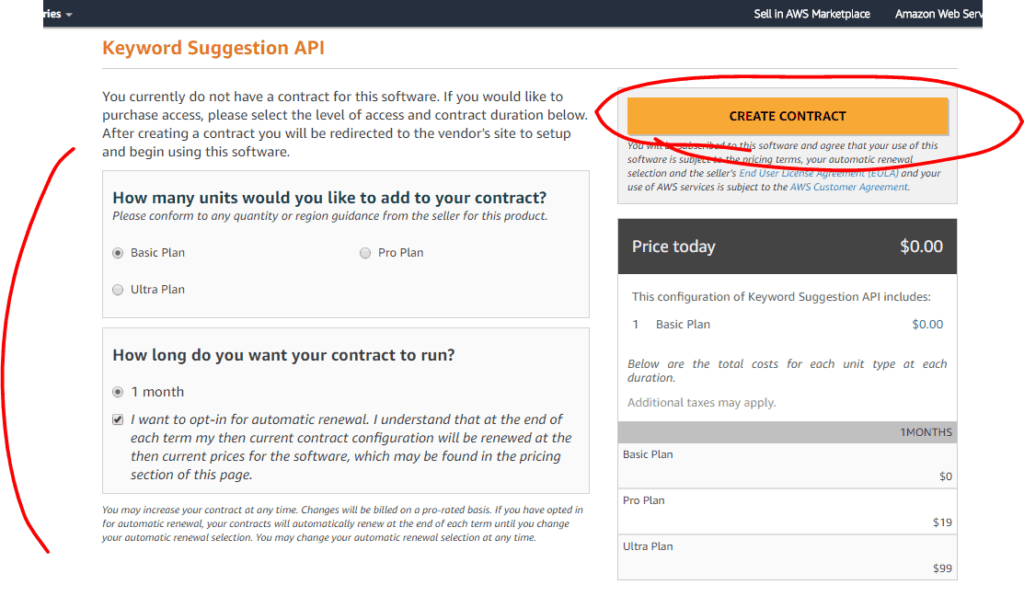This image depicts a user interface for a Keyword Suggestion API, primarily characterized by its orange and gray color scheme. The top left corner of the image includes the header "Keyword Suggestion API" in orange text, with a gray horizontal line directly below it. An orange "Marketplace" header bar is partially visible at the top of the image.

The lower left corner features the abbreviation "RASMR" in uppercase letters, while the lower right corner contains partially visible text reading "Amazon WebServe." A prominent red curved line is on the far left side of the image.

Immediately below the header, a paragraph reads: "You currently don't have a contract for this software. If you would like to purchase access, please select the level of access and contract duration below. After creating a contract, you will be redirected to the vendor site to set up and begin using this software."

Centered in the gray bar above the paragraph, the text asks, "How many units would you like to add to your contract?", followed by three access level options: Basic Plan, Ultra Plan, and Pro Plan. The Basic Plan option is distinguished by a blue circle, while the Ultra Plan and Pro Plan are marked with gray circles.

Below these options, the text prompts, "How long do you want your contract to run?" with a bubble marked for "1 month." Further down and to the right, a yellow-highlighted bar labeled "Create Contract" is circled by superimposed user text. Beneath this is a black bar stating, "Price today is $0," alongside more disclaimer text at the bottom of the image.